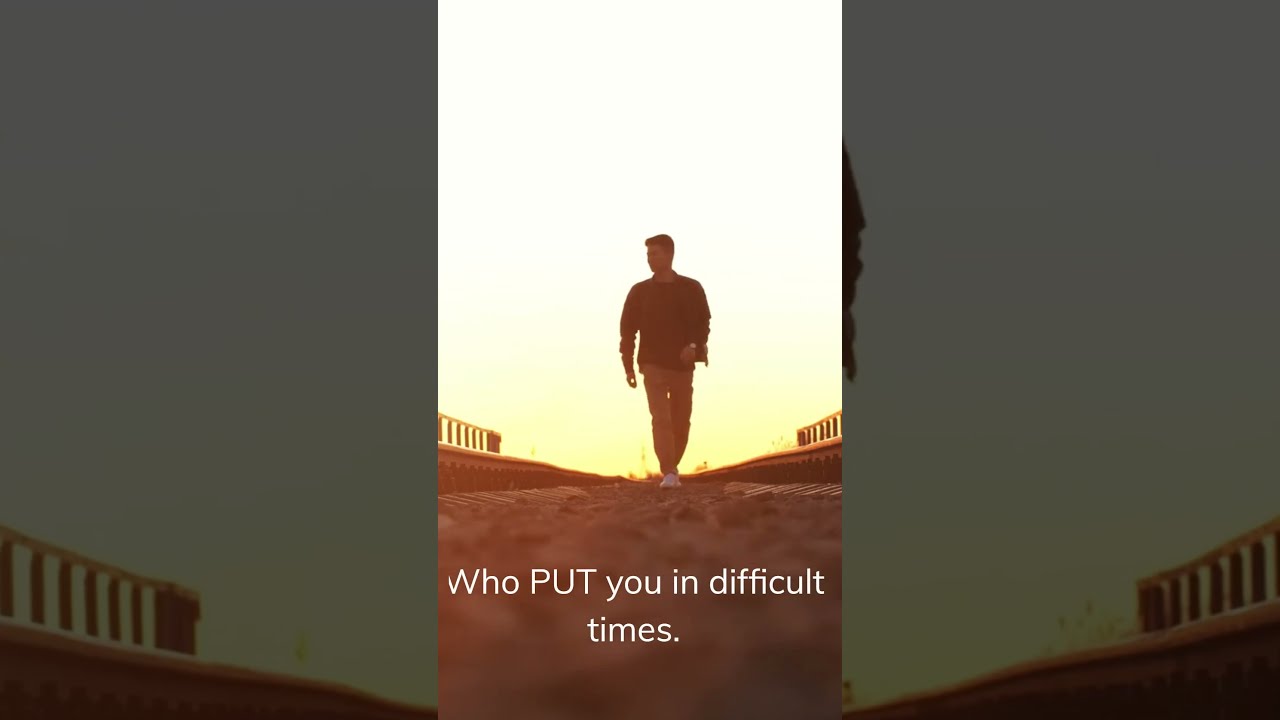The image resembles an illustration with a white background that could be a sky, transitioning to a yellow haze on the horizon, potentially suggesting a sunset. It depicts a man, positioned centrally, walking on what appears to be a railroad track surrounded by railings on each side. The figure, who is slightly angled to his right, wears white tennis shoes, light brown (khaki) pants, a long-sleeved dark shirt, and a watch. The perspective of the photo is from ground level, giving a detailed view of the gravelly path he's on. At the bottom of the image, a caption in white text asks, "Who put you in difficult times?" with the word "PUT" emphasized in all capital letters. Behind the main image, there's a darker, close-up version of the same scene, which provides an additional, albeit less clear, perspective.